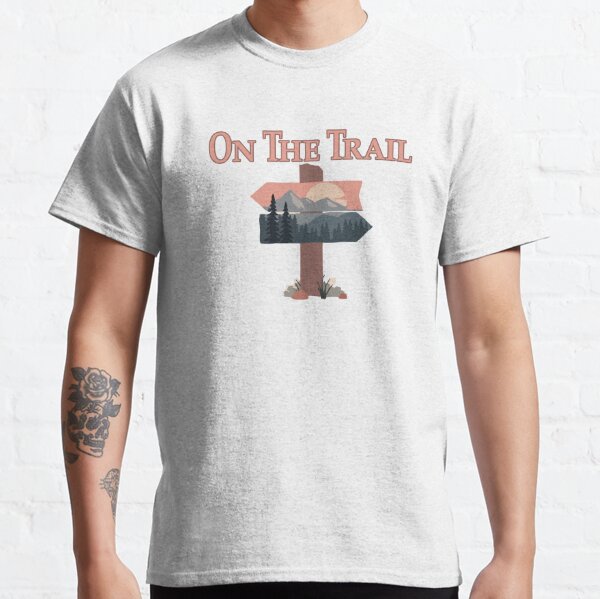The image features a close-up of a white, short-sleeve t-shirt worn by a light-skinned male, showcased against a solid white background. The man has medium skin and a visible tattoo on his right forearm, which appears to wrap around and includes a skull and floral design in green ink. The t-shirt has a central design with text that reads "On the Trail" in cream-colored letters. Below the text, there's an illustration of a wooden post sprouting from the ground, adorned with weeds. The post features two arrows, one pointing left and the other right, and a scenic backdrop that includes a mountain range, pine trees, and a moon. The man's arms are relaxed at his sides, and the lighting enhances the clarity of the image, making the details stand out vividly.